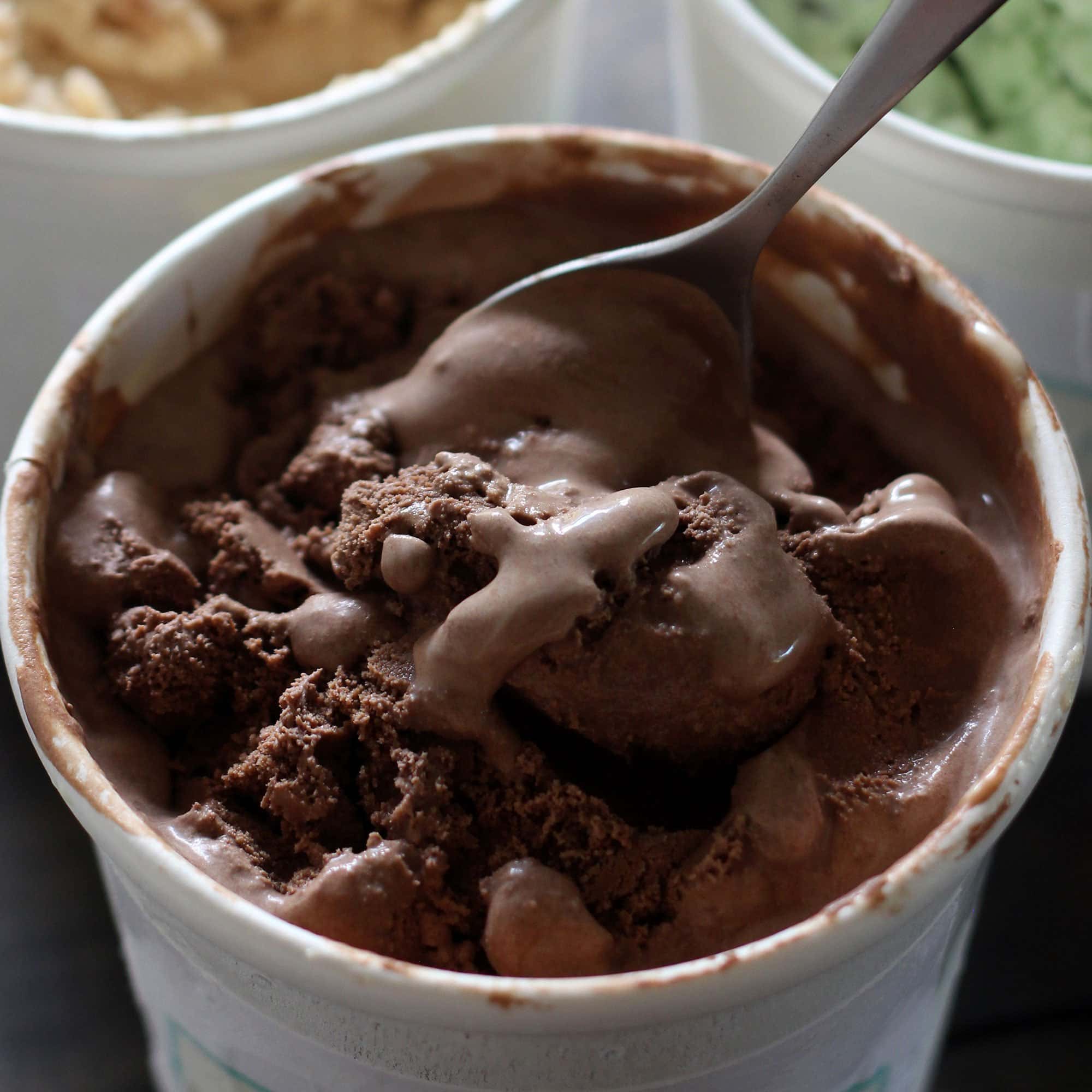A close-up image showcases a pint-sized, white round cup filled with melting chocolate ice cream, placed on a black surface. The chocolate ice cream exhibits a mix of smooth and rough textures, with some areas appearing muddy and clumped. A silver spoon is inserted into the ice cream, with its handle sticking out prominently. Chocolate is smeared all over the container's messy rim. In the top left and right corners of the image, there are partial views of additional white cups containing what appears to be yellow and green ice creams, likely vanilla and mint, though the details are slightly faded. This emphasizes a scene of indulgent, slightly messy enjoyment.